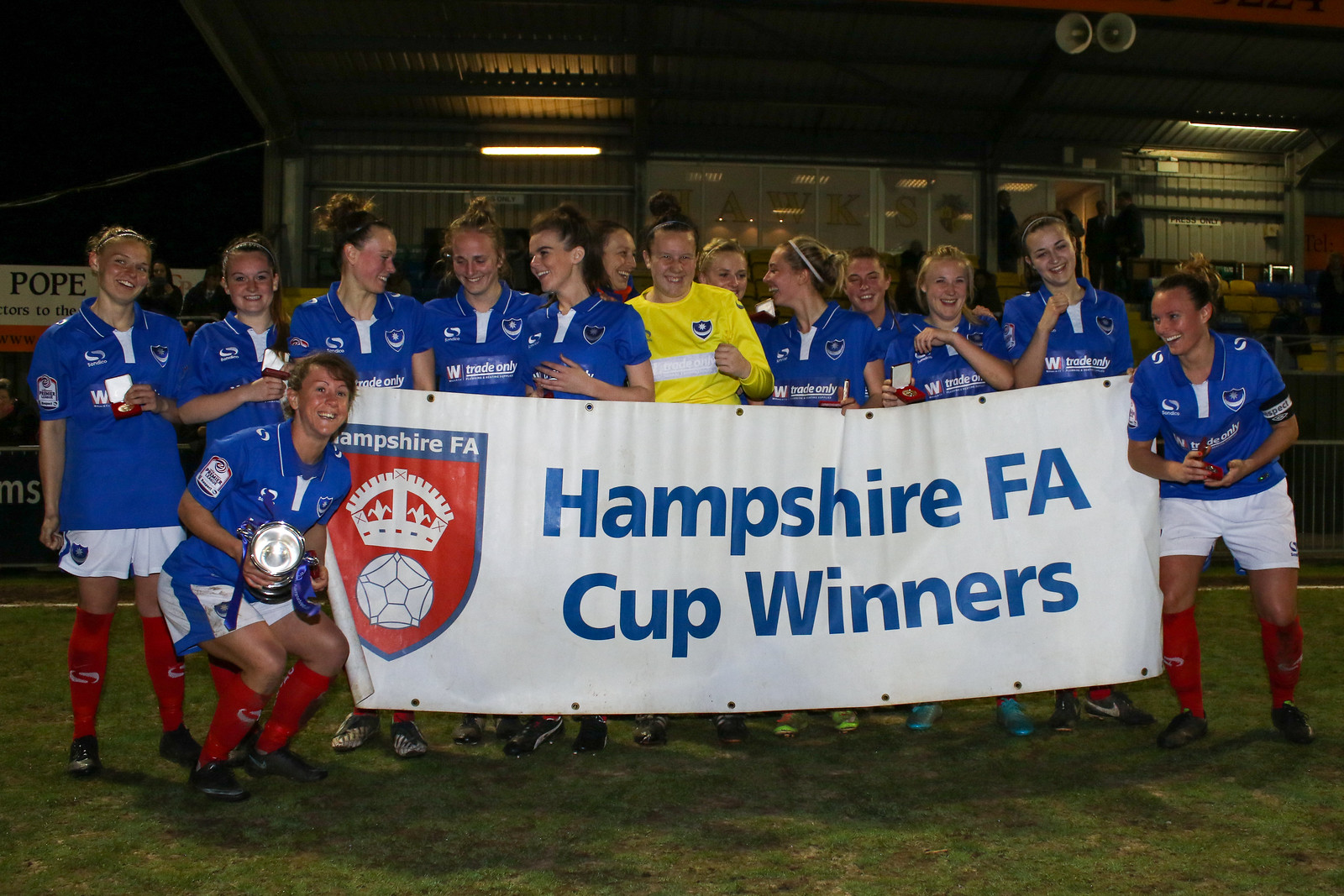In the photograph, we see a jubilant group of 14 college female athletes standing on a soccer field at night, with smiles lighting up their faces. Their team uniforms consist of bright blue jerseys, white shorts, and knee-high red socks, complemented by various soccer cleats. The majority of the women have their hair neatly tied in buns, and they appear tanned and uniformly Caucasian. The central figure, likely the goalie, stands out in a yellow outfit amid the sea of blue.

The team is holding a large banner that reads "Hampshire FA Cup winners" in bold blue text on a white background, adorned with a shield featuring a crown and a soccer ball on the left side. Additionally, some of the athletes proudly hold up trophies, with the player in the front left prominently displaying a larger trophy.

Illuminated by a light source behind them, which casts a glow on their happy faces, the photograph is taken against a backdrop that reveals parts of a building, perhaps on their school grounds, and a fence with advertisements, though their texts are not legible.